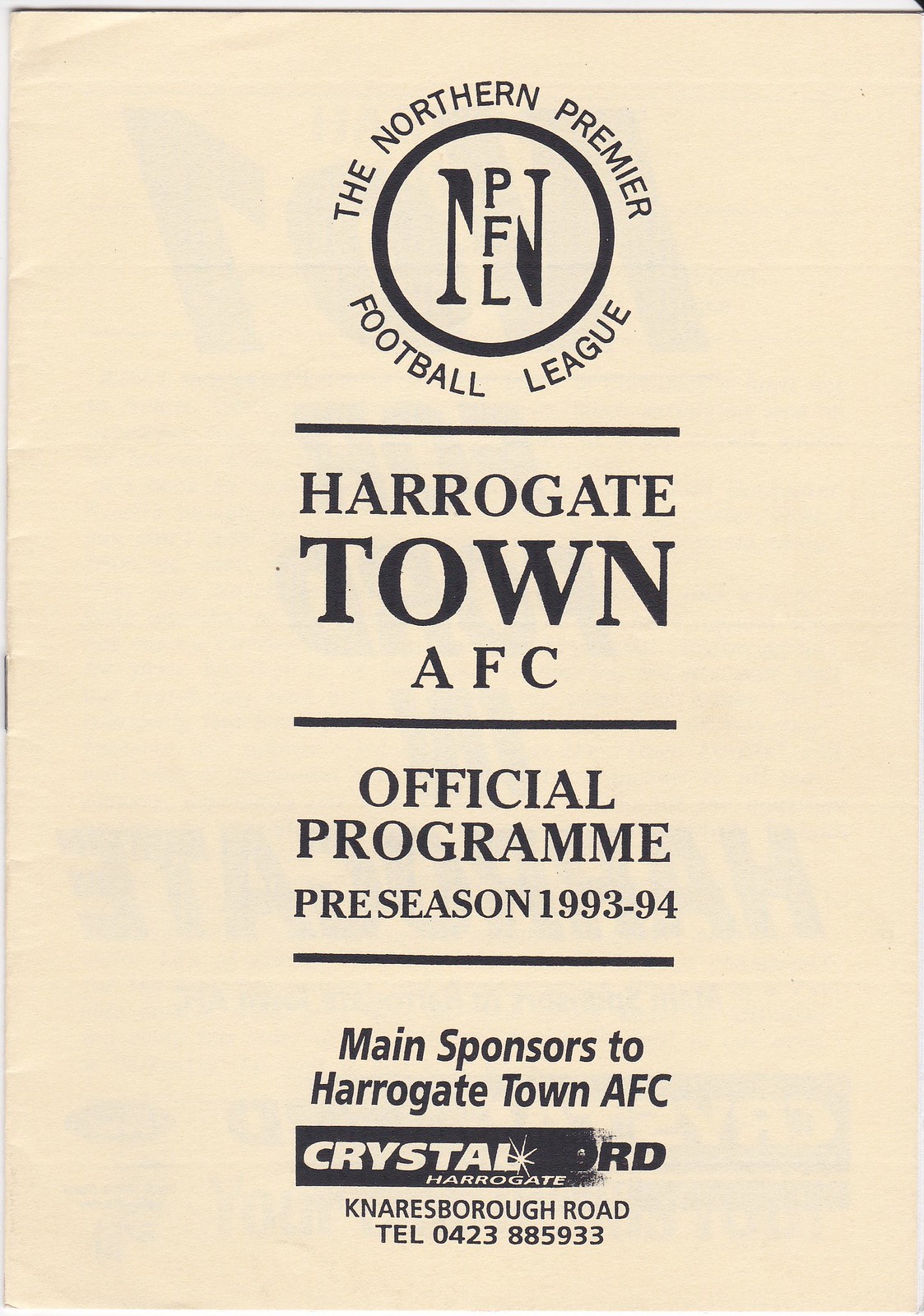The image depicts an official program booklet for the Harrogate Town AFC, associated with the Northern Premier Football League, for the preseason of 1993-1994. The booklet features a prominently displayed heading in black text that reads "Northern Premier Football League" at the top, followed by "Harrogate Town AFC Official Program Preseason 1993-1994." The main sponsor, Crystal Harrogate, is highlighted below with their logo, which includes a star and is written in capital letters. Additionally, the sponsor's contact details are provided: Naresboro Road, Telephone 0423-885-933. The entire booklet, which appears old and somewhat beige from age, is likely stapled on one side, suggesting it was meant for easy flipping through. The text and overall design, centered within the pale tan background, give it a vintage, newspaper-like aesthetic, with some faint, faded imagery of other pages visible beneath the main text.